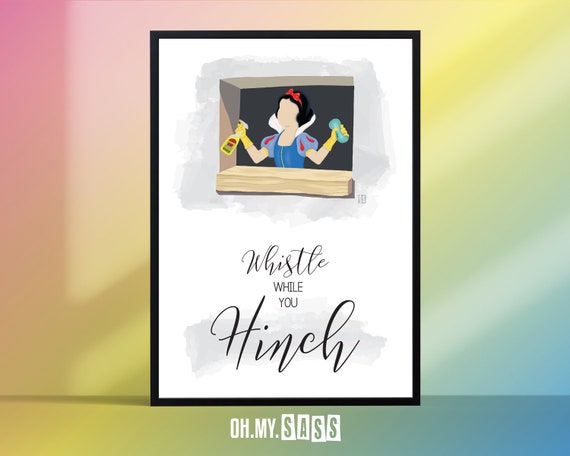The image depicts a vibrant, rainbow-colored diagonal gradient background, transitioning through blue, yellow, red, pink, green, and blue hues. Positioned against this colorful backdrop is a seemingly illustrated poster with a black border and white background, giving the impression of being physically propped up but likely crafted in an art program due to its unrealistic shadow.

At the top of the poster, there is a stylized, faceless cartoon character resembling Disney’s Snow White, clad in her iconic blue dress with a red ribbon, though faceless. She is depicted holding a cleaning sponge in one hand and a can of cleaner in the other, while wearing yellow gloves. The character is positioned in front of a small window.

Below this illustration, cursive and print lettering reads, "Whistle While You Hinch," suggesting a whimsical twist on the classic "Whistle While You Work" theme from Snow White. Further down, below the poster's edge, additional text spells out, "OH. MY. SASS," with the word "sass" encased in individual squares, indicating possible brand or stylistic choice in the design.